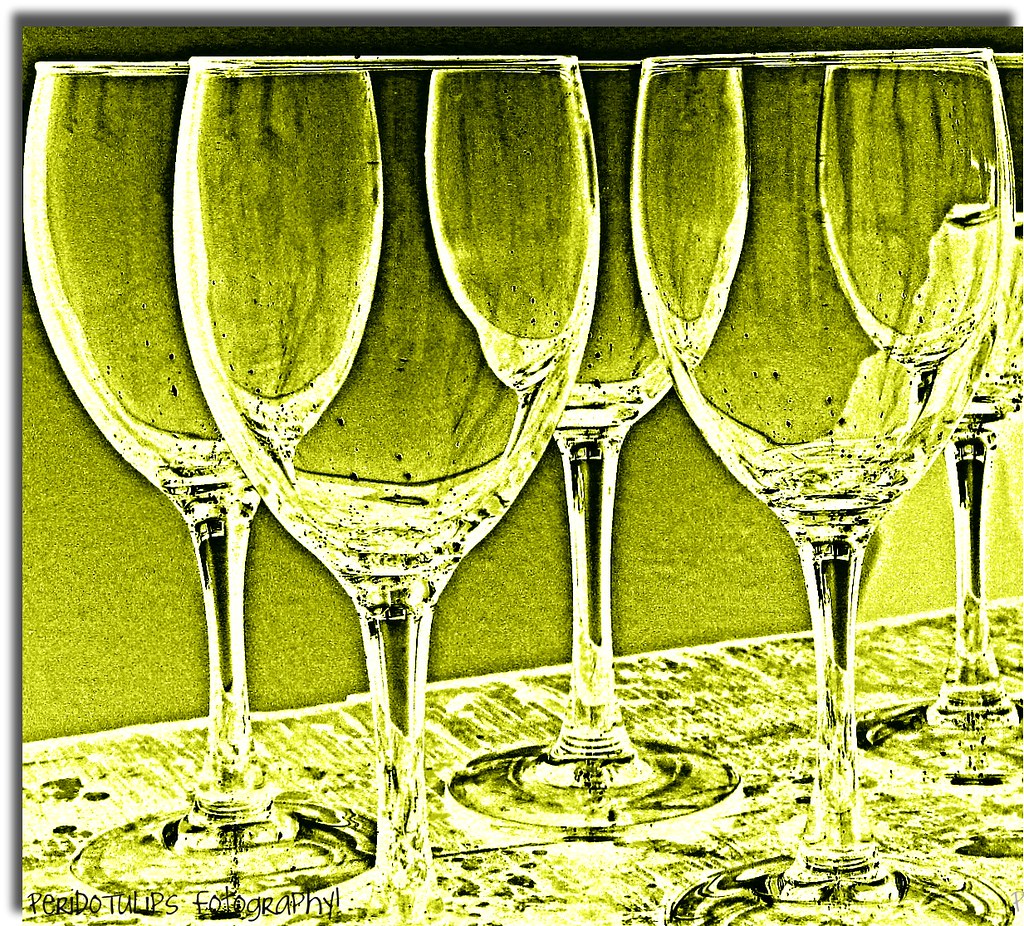The image features five stemmed wine glasses, possibly crystal, arranged on a textured surface. The photo has been heavily edited, giving it a green filter that washes out most of the detail and creates a swampy, high-contrast effect. Two of the glasses are positioned in the foreground, with three more behind them, partially visible through the transparent material of the foremost glasses. This layered arrangement results in an intricate pattern of overlapping, half-visible spheres. In the bottom left corner, the text "Perito Tulips Photography" is visible, though "Photography" is misspelled as "FOTO". The distorted filter and altered coloring, which includes tones of yellow, black, and white, suggest an artistic or experimental approach, possibly a marketing piece or practice work for the photography studio.